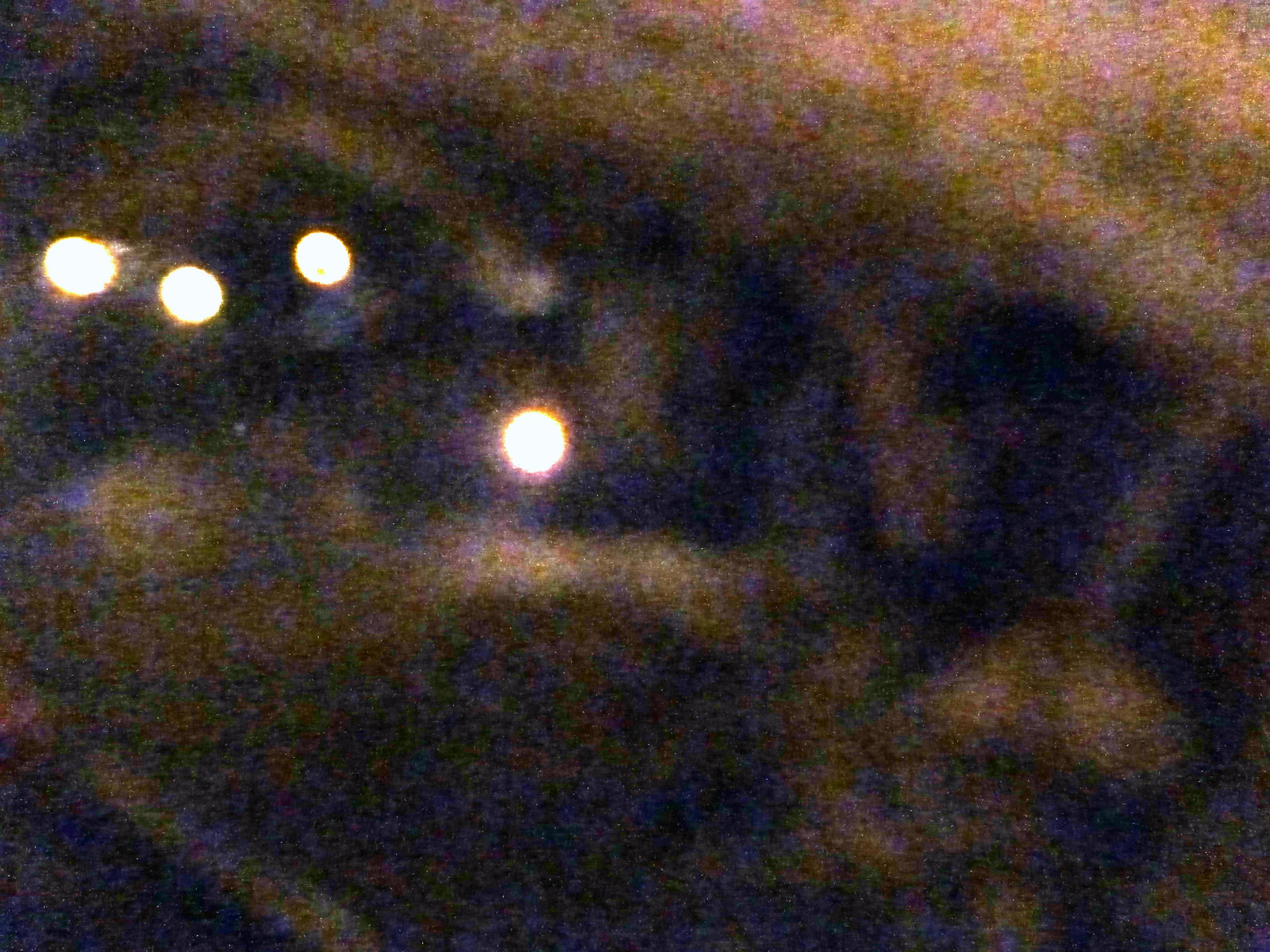This image is exceedingly blurry and out of focus, rendering the subject almost entirely unidentifiable. The primary visible elements are four small, round lights. Three of these lights are clustered closely together in the upper left section of the image, while the fourth light is positioned slightly down and to the right toward the middle of the frame. Due to the extreme lack of clarity, it is difficult to determine whether these lights are actual objects or simply reflections. The photograph is marred by indistinct light and dark patches scattered throughout, suggesting potential issues with either the developing process, digital processing errors, or possible obstruction of the camera lens. Overall, the poor quality of the image makes it impossible to discern any clear details.